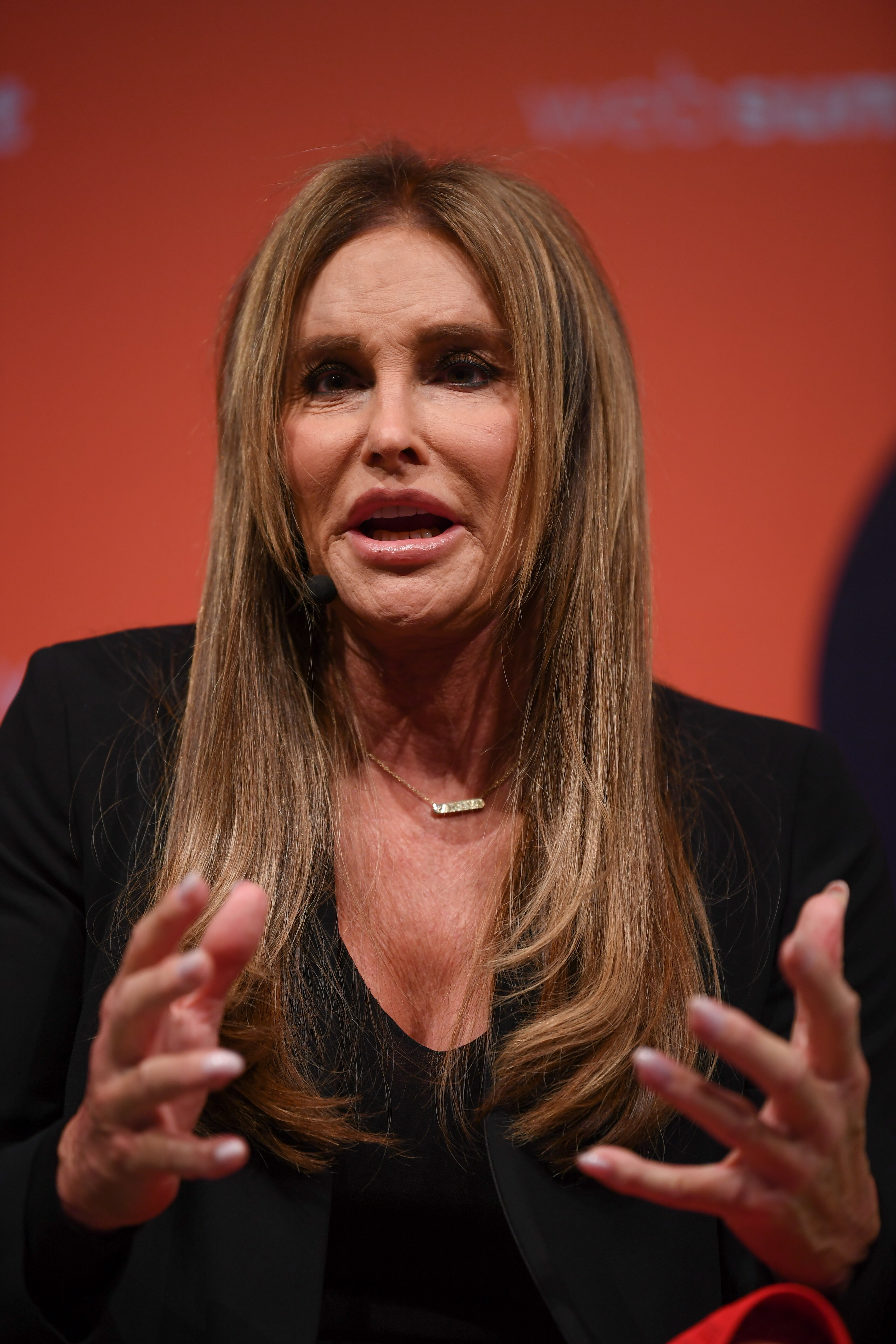This vertically aligned rectangular image captures an elderly woman at a conference, who appears to be an actress or news broadcaster. She is the focal point of the photograph, standing out against a blurred orange background with some white lettering and indistinct blueprints in the upper corners. Her long, light brown hair is parted in the center and cascades over both shoulders. The woman's skin is tan, and she appears to have had cosmetic surgery on her lips, which are partly open to reveal her teeth. Deep wrinkles are visible on her chin, forehead, and under her eyes, though her eyes themselves are in shadow. She is dressed in a low-cut black shirt with a black business jacket over it, complemented by a gold chain necklace adorned with rectangular pendants close to her neck. She has unpainted, long fingernails and is gesturing with her hands in front of her, likely speaking. In the lower right-hand corner of the image, a red strap or object is visible, though it is unclear what it is.